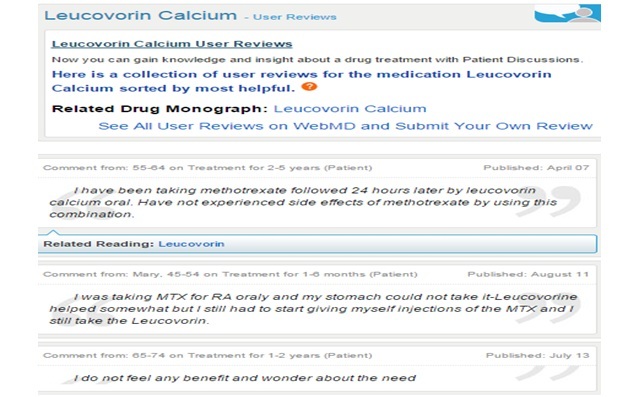**Detailed Descriptive Caption:**

A screenshot of a webpage titled "Luther Corvin Calcium User Reviews" features prominently. To the right of the title, an image of a person appears, with a speech bubble emanating from their mouth, indicating a verbal communication. The speech bubble reads "Luther Corvin Calcium User Reviews," emphasizing the focus on patient discussions about the drug treatment. The webpage offers the promise of gaining knowledge and insights through a collection of user reviews on Luther Corvin Calcium, sorted by the "Most Helpful" category. 

An orange circle with a question mark is visible, possibly indicating a help or informational section. Below it, the text "Related Drug Monograph: Luther Corvin Calcium" is displayed, along with a prompt to see all user reviews on WebMD and submit personal reviews.

In the review section, a highlighted box contains a patient's experience: "I've been taking methotrexate followed two to four hours later by Luther Calcium oral. I have not experienced the side effects of methotrexate by using this combination." 

Following this, another review states: "I took it orally, and my stomach could not take it," highlighting adverse reactions. A third review expresses dissatisfaction: "I do not feel any benefit and wonder about the need." The reviews are timestamped with dates indicating their publication: July 13th, August 11th, and April 7th, giving a timeline of user experiences.